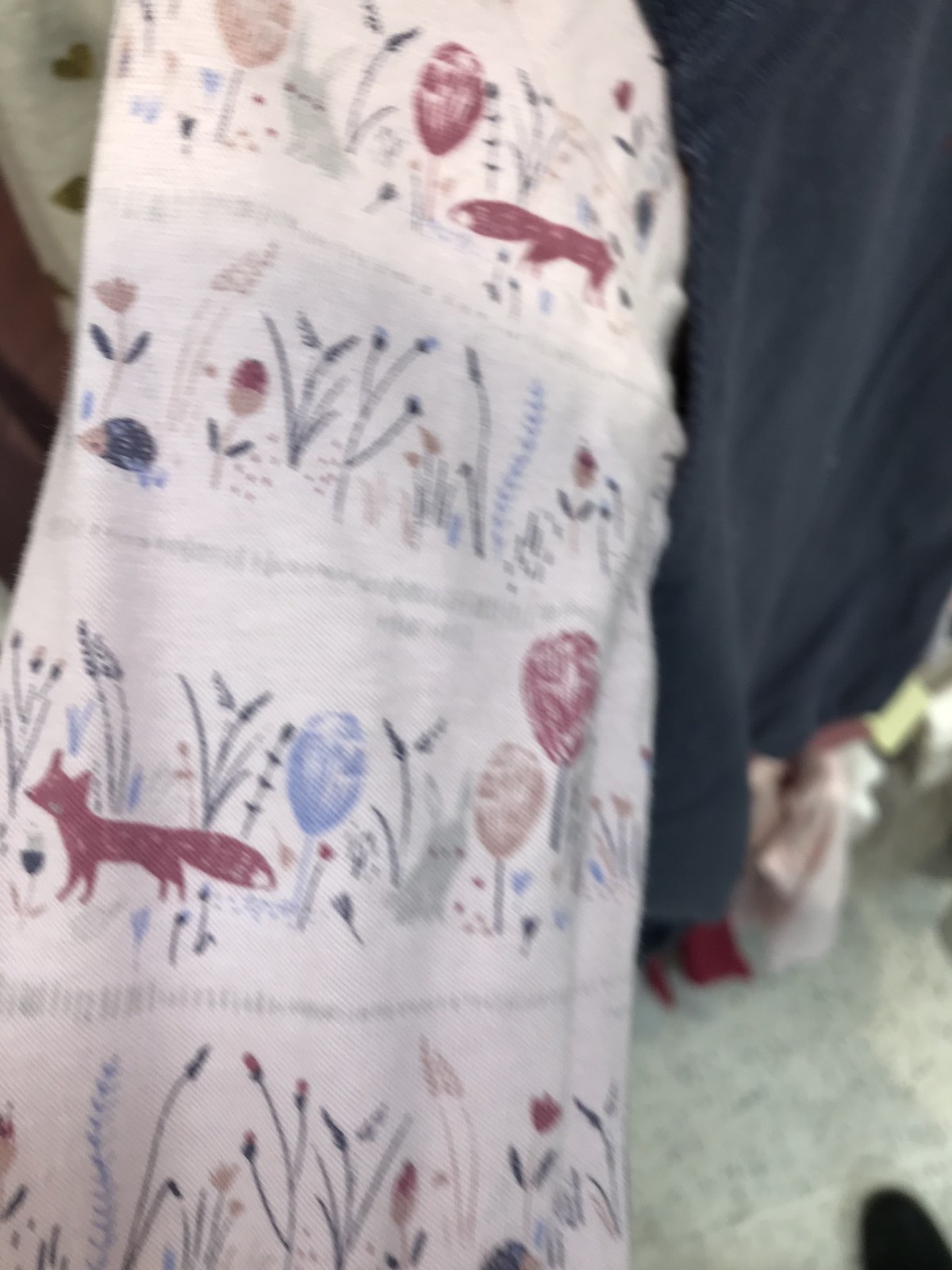A beautifully crafted piece, this image showcases what appears to be a delicate, possibly handmade scarf or a section of a duvet. The fabric is a soft, pastel pink adorned with whimsical drawings. Four horizontal sections, divided by light green lines, each feature unique artwork. Starting at the top, a charming fox graces the first section. The second section depicts what seems to be a porcupine amidst some delicate floral designs. Another fox appears in the third section, equally enchanting. The final part is dedicated entirely to intricate floral illustrations. The light and playful imagery, coupled with the soft color palette, gives this piece a dreamy, handcrafted aesthetic.